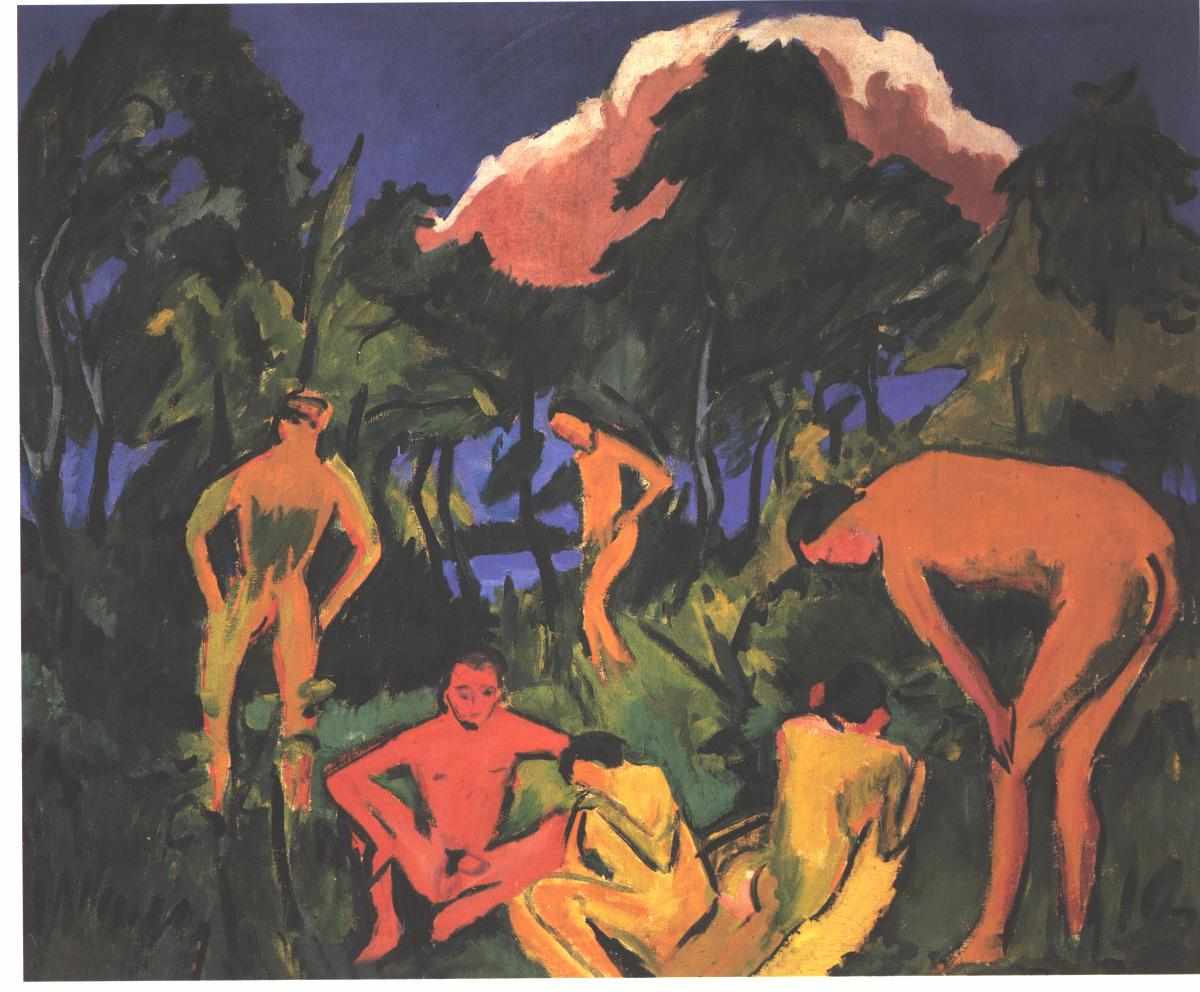This horizontal-rectangular abstract painting features a dark, lush forest scene where six nude figures, diverse in both positioning and color, are present. The background sky is a dark purple, contributing to the overall dim ambiance. Two yellow figures sit in the front; one is bent over and possibly a woman, and the other has his back to viewers. To the left, a reddish-orange man sits cross-legged, exposing his genitals. A man on the bottom right corner stands, leaning over, and is orange, revealing his butt crack. Another seated figure, colored light shade of orange, turns away from the viewer towards a tree. Additional figures are scattered, blending into the vibrant green grass and foliage. Above them, two orangey clouds, vaguely human-shaped, float in the night sky, adding a surreal touch to this summertime forest scene.